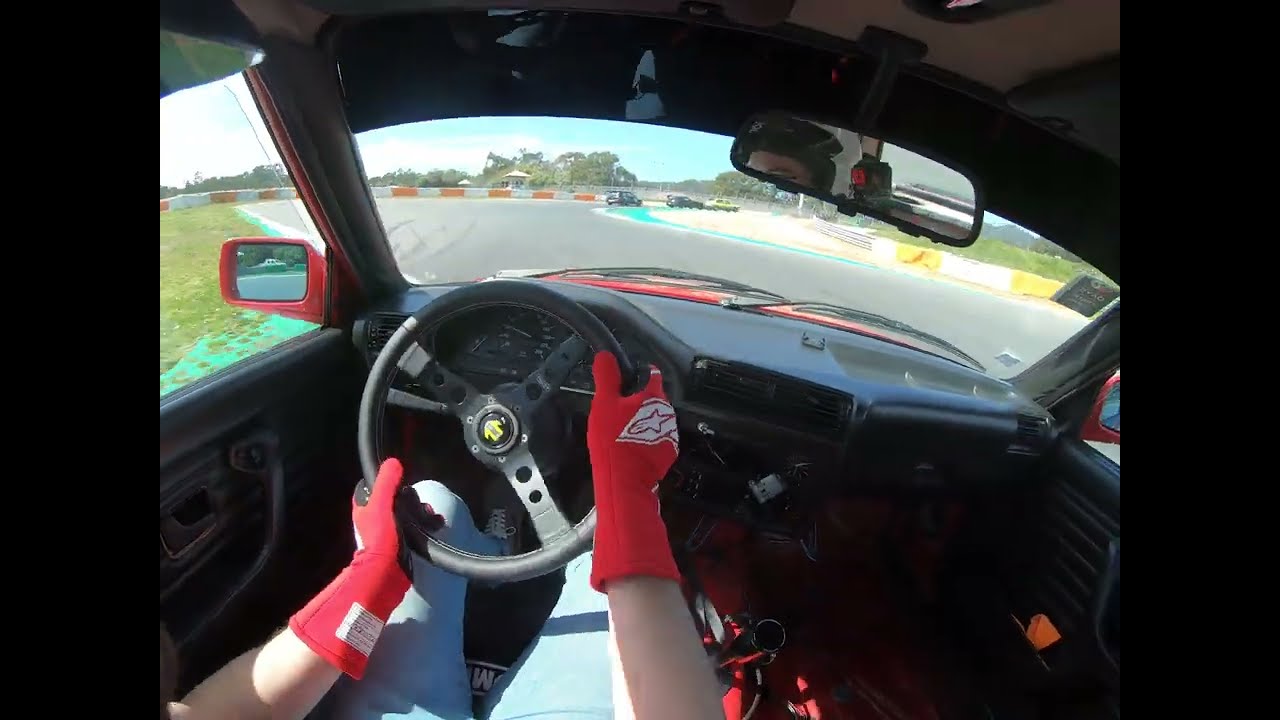The image is a dynamic, first-person perspective captured from a GoPro-style camera mounted on the driver's head, immersing us in the experience of driving what appears to be a race or rally car, given the detailed context. The driver, with light-toned skin, is wearing red gloves—possibly driving or winter gloves—that have white accents. Their left hand grips the lower part of the black steering wheel, which features a yellow insignia in its center, while their right hand is positioned near the middle, indicating they are navigating a right curve in the road. They are dressed in blue jeans, and a hint of a beanie is visible, suggesting that's their headgear.

The interior of the car is primarily black and red, including the dashboard and hood, with a red side view mirror visible. There’s a small rearview mirror hanging above, and some additional red detailing is present lower center inside the vehicle. The car itself lacks a passenger seat, reinforcing the notion it's designed for racing.

Outside the vehicle, the scene is set on a curving paved road under a bright blue sky. To the right of the vehicle, there's a yellow and orange-striped barricade, alongside some sandy patches and a grassy infield, implying the setting is more rural or country-like. In the distance, a white and orange makeshift guardrail, along with some trees, are noticeable. A few other cars can be seen navigating the same curve ahead, further emphasizing the sense of movement and speed. The left side window reveals more grass, adding to the rural ambiance, while the overall condition of the car appears well-maintained.